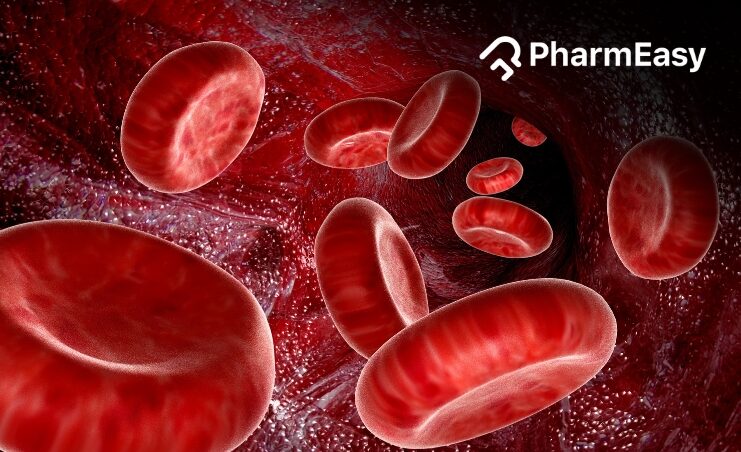The image depicts an artistic rendition of red blood cells within an artery. The backdrop is a deep red, with fleshy-looking walls speckled with white dots, simulating the texture and flow within a blood vessel. Scattered throughout the image are about ten red blood cells, each appearing at different orientations—some lying flat, others slightly curled—creating a dynamic sense of movement. The cells vary in size, appearing larger in the foreground and shrinking with distance, adding depth to the scene. A distinctive white outline edges each cell, enhancing their visibility against the red background. Positioned at the top right corner, the text "Farm Easy" is displayed in a white font. Notably, a small curvy symbol resembling a stylized design is located near the text.